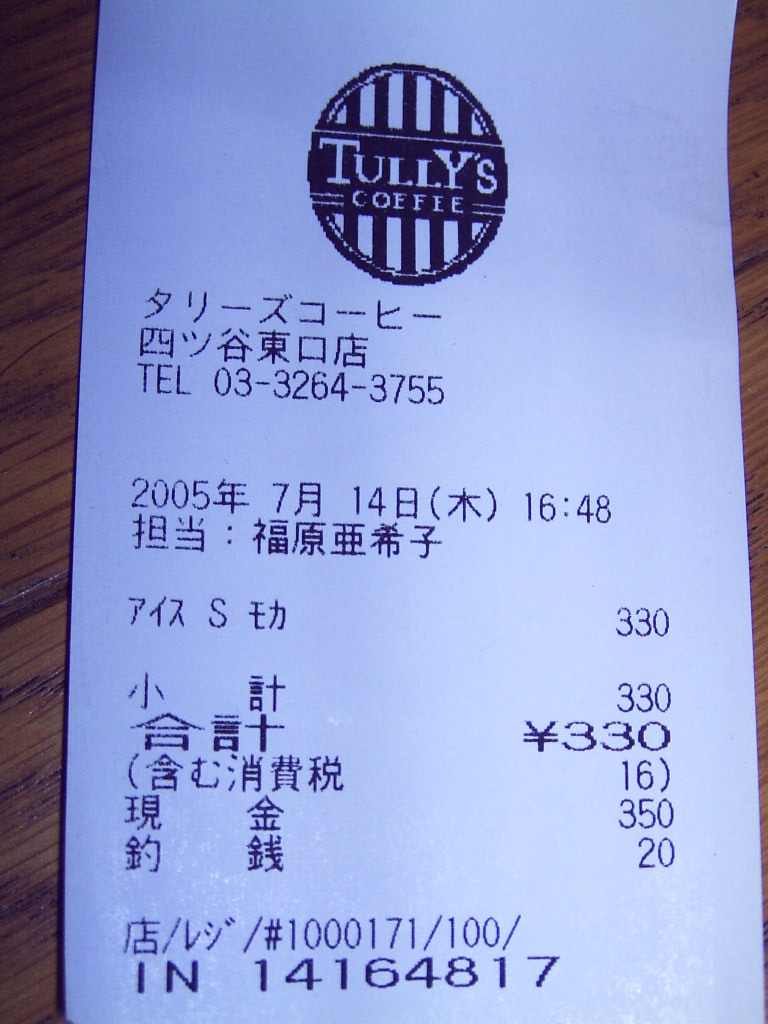The color photograph features a white receipt from Tully's Coffee, prominently displayed on a dark mahogany wooden surface, with the planks running slightly diagonally from left to right. At the top of the receipt is the Tully's Coffee logo, a black circle with vertical black and white stripes, and a horizontal black banner across the circle with white letters spelling "TULLY'S Coffee." The majority of the text on the receipt is in traditional Japanese characters. Key details include a telephone number, 03-3264-3755, and a date and time stamp, 2005-7-14 16:48. The receipt shows several numeric entries: ¥330 appears in connection with both the amount paid and some other entries, while ¥350 is listed further down without a yen symbol next to it. Additional notes include the invoice number 14164817 and other numeric values such as 16 and 20.